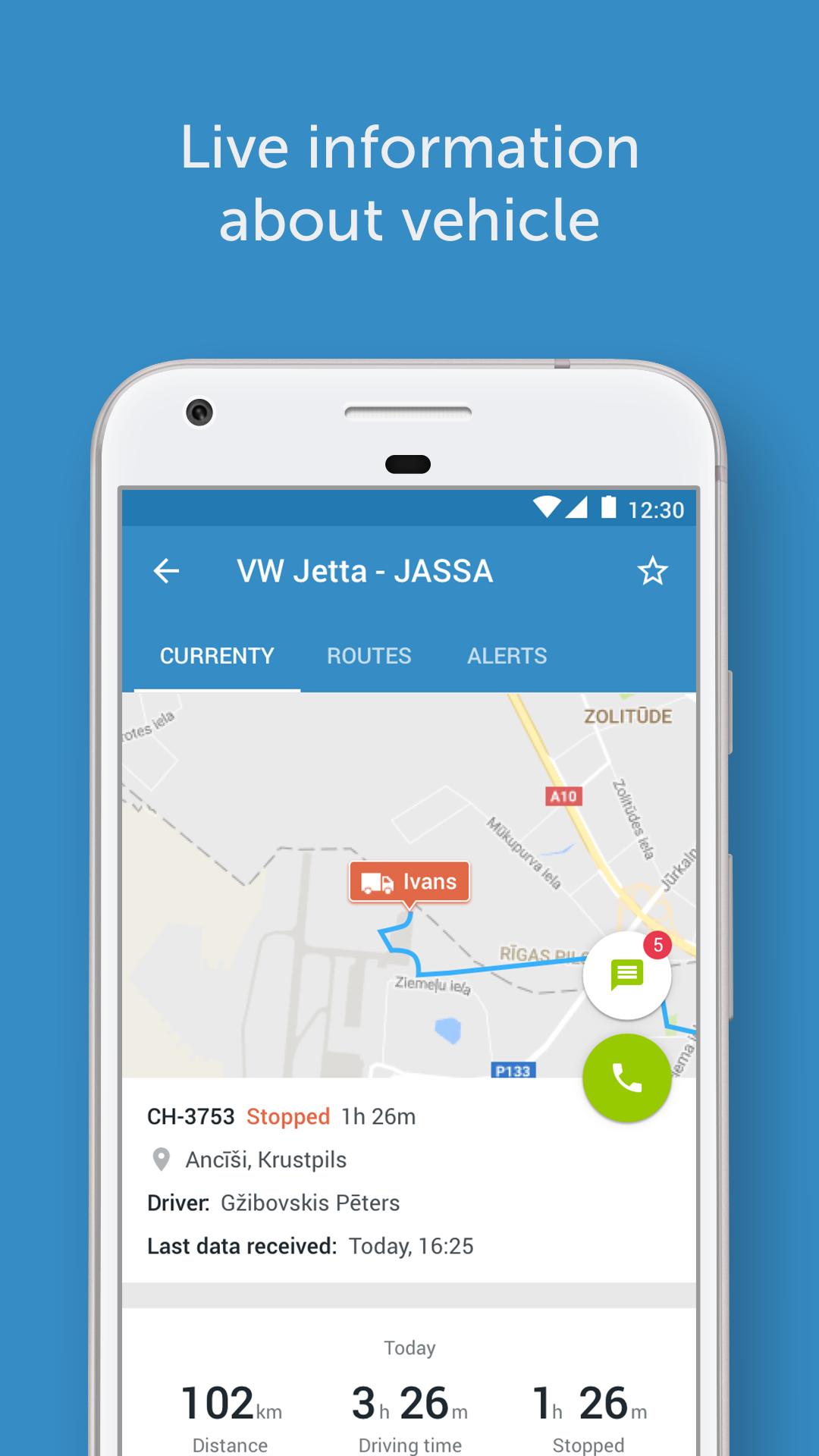Detailed Caption: 

The image depicts an advertisement for a mobile application against a blue background. Prominently displayed at the top in large white font is the phrase "Live Information About Vehicle." Below, a mobile device is showcased, featuring a camera positioned in the upper left-hand corner and a visible speaker at the top, indicating this is a real screenshot of the app interface on the phone. The mobile device, appearing predominantly white, shows typical indicators such as the carrier signal and battery life. The time displayed on the phone is 12:30.

The application interface displayed on the mobile screen focuses on a Volkswagen Jetta with the identifier JASA. Key sections of the app include "Currently," "Routes," and "Alerts." Additionally, there is a prominent favorite button represented by a star icon at the top of the screen. A map is visible within the app, and details such as "CH3753, stopped 1 hour and 26 minutes" are listed. An orange button labeled "Ivan's" with a truck icon is highlighted. Further information includes the driver’s name and the last data received today at 16:25.